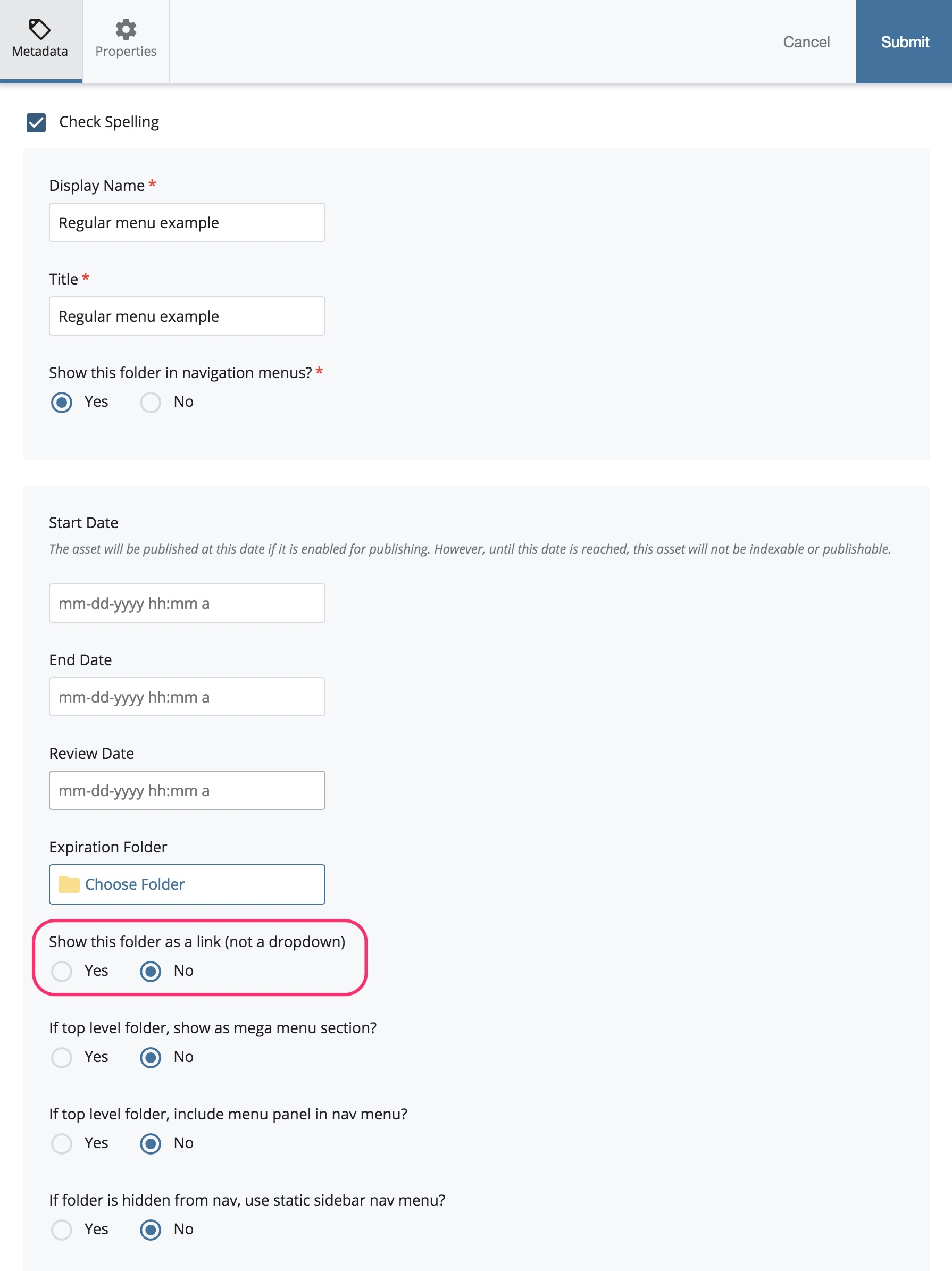This screen capture displays a user interface for managing metadata and properties of a digital asset. At the top, a banner includes highlighted and non-highlighted square icons: one for "Metadata" with a tag symbol and another for "Properties" with a gear symbol. On the right side of the banner are the "Cancel" and "Submit" buttons, with "Submit" highlighted in blue.

Below the banner, a blue-checked checkbox for the "Check Spelling" option is visible. The gray-background dialog box beneath this contains a field labeled "Display Name" marked with a red asterisk indicating it's required. The field is populated with "Regular Menu Example."

Further down, another required field with a red asterisk includes options for showing a folder in navigation menus. It contains radio buttons for "Yes" and "No," with "Yes" currently selected.

A second dialog box with a light gray background is dedicated to the "Start Date." It mentions that the asset will be published from this date if enabled and emphasizes that until this date is reached, the asset will not be indexable or publishable. This section also includes text entry boxes for input.

Overall, the layout provides a detailed and organized approach to managing digital assets' settings.